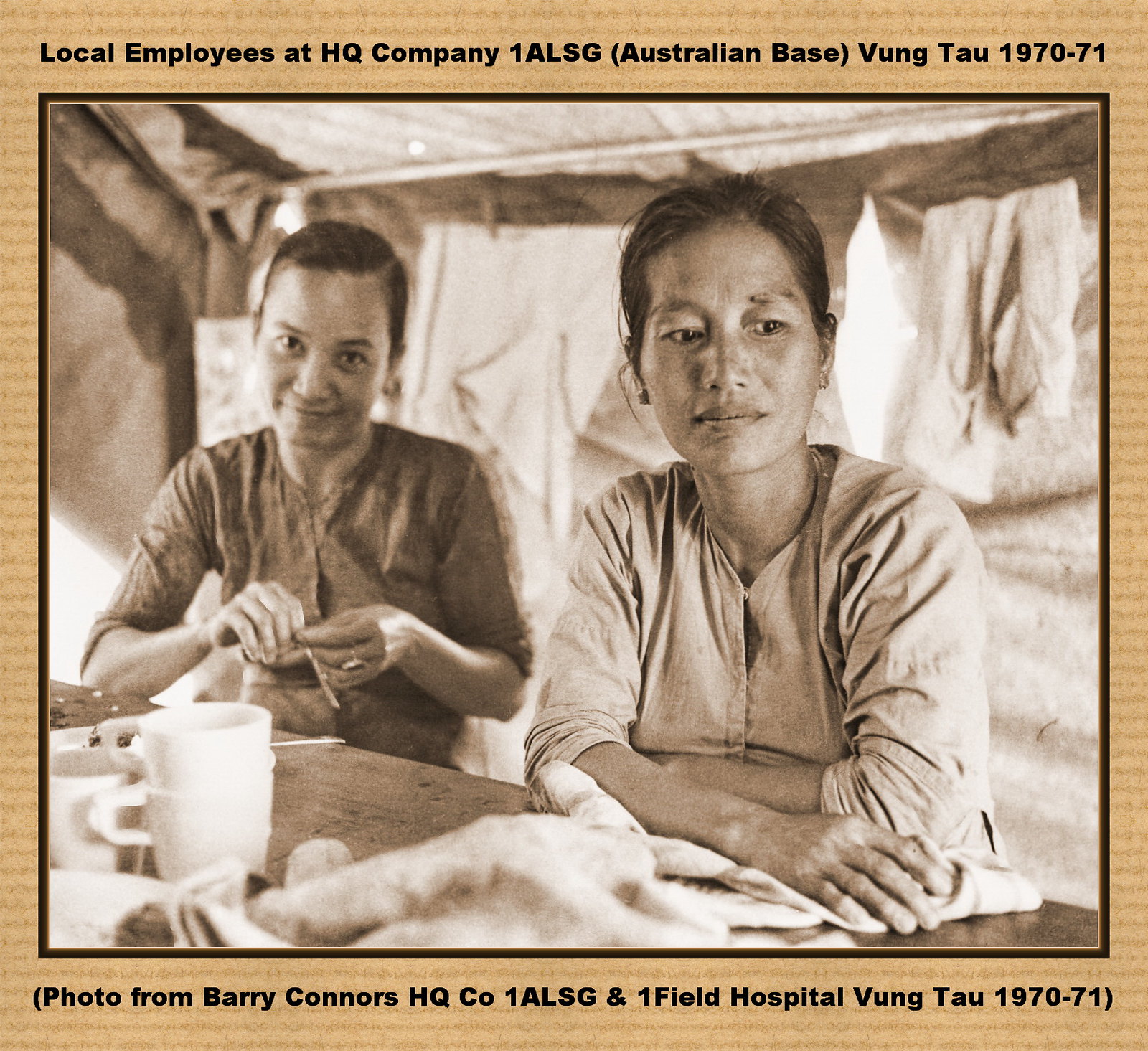This historical black-and-white photograph captures a poignant moment at the Australian Base, HQ Company 1ALSG in Vung Tau, Vietnam during 1970-1971. The image, taken by Barry Connors, features two female employees seated at a table, possibly taking a break from their work. The woman on the left, with short dark hair and a slight smile, looks directly at the camera with her hands poised above the table. Her counterpart, on the right, has her dark hair pulled back, gazes off to her right with a serene smile, and rests her folded hands on the table. Both women wear rolled-up long-sleeved shirts, and the table in front of them holds three white mugs, two of which are nested together. The photo is set against a light brown background, likely indicative of its use in a museum or historical publication, and provides a glimpse into the everyday lives of those who served during the Vietnam War. Text above the photo identifies the location and date, while text below attributes the photograph to Barry Connors.